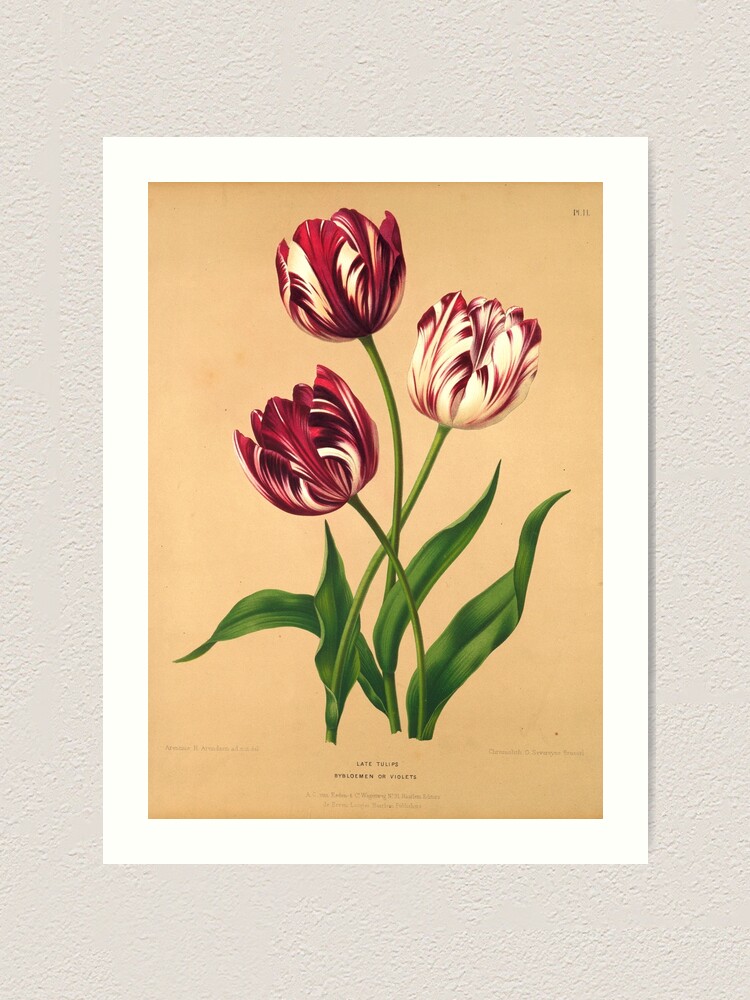This detailed painting features three vibrant tulips, each with lush green leaves and intertwined stems, set against a light orange, almost peach-colored background. The whole artwork is framed by a clean white border and positioned on an off-white wall. The tulips, known as Rembrandt tulips, exhibit a captivating "candy stripe" effect due to a unique virus, blending striking red and white hues.

The tulip on the far right is predominantly white with subtle touches of dark red, giving it a delicate appearance. In contrast, the two tulips on the left and in the center showcase deeper, maroonish-red petals with white accents. The leaves are notably long and thin, resembling wide strands of grass.

The painting is rectangular, taller than it is wide, and has some small, black-font text beneath the flowers that reads "late tulips," though the rest is too tiny to discern. The overall image is a beautiful and healthy depiction of tulips, thoughtfully capturing the intricate details and colors of these striking flowers.